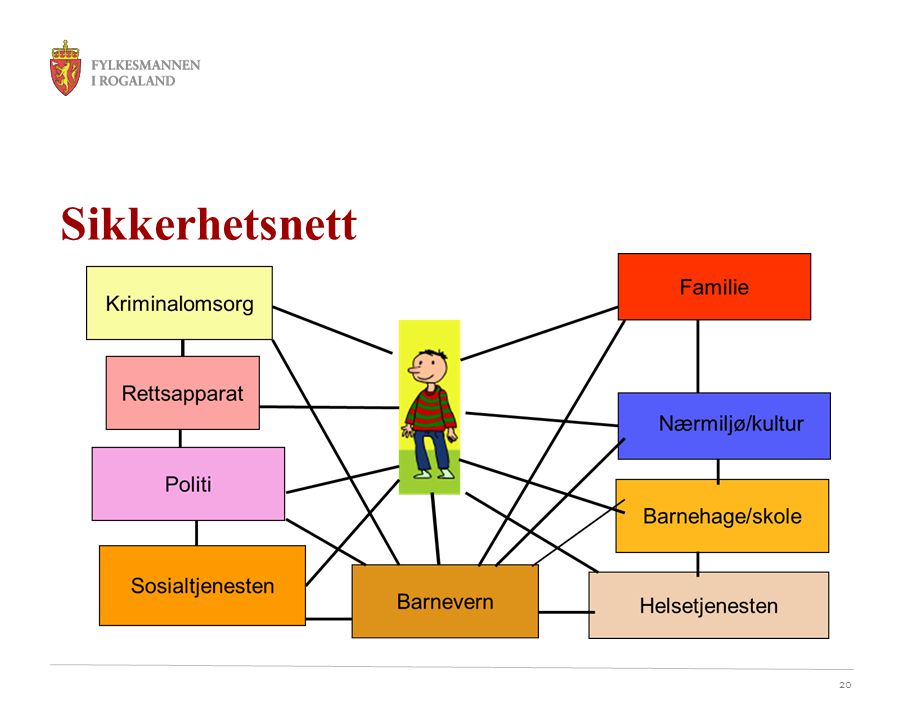The image features a detailed computer-generated diagram set against a white background. Predominantly occupying the top left corner is a yellow shield icon, resembling a university logo, adjacent to the text "Faiql's Manan-i-Ragaland" or "Falkasman Rogaland." Below this, in red text, reads "Sikr Het Snet" or "Seeker Heads Net." Central to the image is a cartoon figure of a boy standing, surrounded by numerous rectangular boxes of various colors, each containing different words that appear to be translations or variations of similar concepts, potentially in different languages.

These boxes are connected both to the boy and to each other with lines, forming an intricate network. Specifically, there are four boxes on the left side of the figure, four on the right, and one directly below. Notable boxes include a yellow box with a black border labeled "Kriminalam Sorg," a pink box with a black border labeled "Ret Sa Parat," and a pinkish-purplish box with a black border labeled "Politi." The colors of the boxes range from yellow, pink, purple, red, blue, tan, beige, brown, to green, making the diagram visually engaging. The overall layout suggests a thematic connection between the boy and the words surrounding him, implying that these words might be interpretations or translations related to the boy's context.